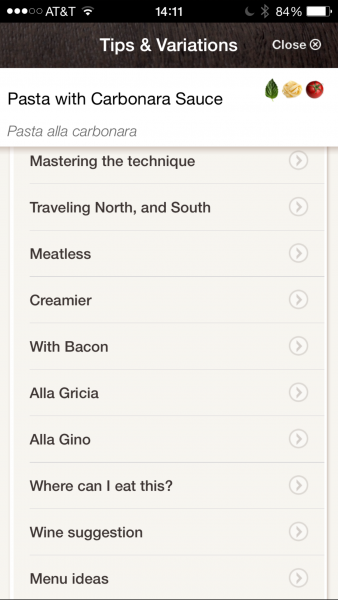The screenshot features a smartphone interface with numerous elements. At the top, within a black status bar, there are five circles, three of which are illuminated white. The status bar displays "AT&T," two Wi-Fi bars, a clock showing 14:11, an inactive quarter moon icon, an inactive Bluetooth icon, and a battery indicator at 84%.

Beneath the status bar is a dark gray block extending across the width of the screen, with the text "Tips and Variations" in white on the left and a "Close" option symbolized by an "X" inside a circle on the right.

Further down, there's a white area featuring an image of a green leaf, garlic, and tomato, accompanied by the text "Pasta with Carbonara Sauce" in black font. Underneath this, there is a line of italicized gray text reading "Pasta Alla Carbonara."

Following this, a large, off-white section is filled with black text. At the top of this section, "Mastering the Technique" is written, followed by a right-facing arrow inside a circle, and a series of topics each separated by a gray line. The topics listed are:

- Traveling North and South
- Meatless
- Premier
- With Bacon
- Alla Gricia
- Where Can I Eat This?
- Wine Suggestion
- Menu Ideas

Each topic is accompanied by a right-facing arrow inside a circle, indicating clickable or expandable options. The detailed layout and information guide the user through various aspects of mastering carbonara sauce and its variations.